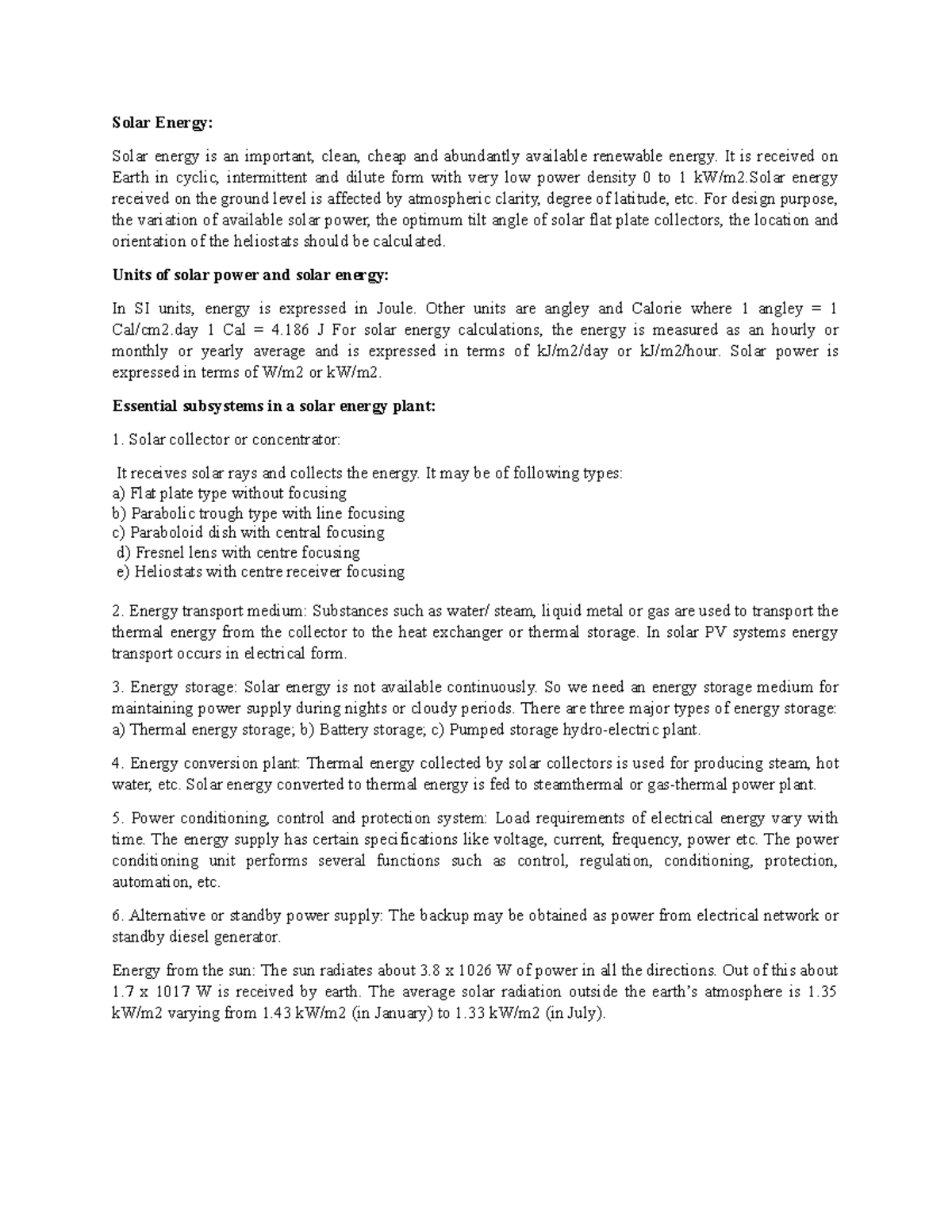This screenshot captures an article dissected into several informative sections, each introduced by bold headings. The sections include "Solar Energy," "Units of Solar Power and Solar Energy," and "Essential Subsystems in Solar Energy Plan." 

The introductory paragraph emphasizes the significance of solar energy, categorizing it as a vital, clean, economical, and abundantly accessible renewable resource. It highlights the cyclic, intermittent, and dilute nature of solar energy received on Earth, which typically exhibits a low power density ranging from 0 to 1 kilowatts per square meter. The narrative stresses how the intensity of solar energy at ground level is influenced by factors such as atmospheric clarity and latitude. 

For design optimization, the paragraph advises calculating variables such as the variation in available solar power, the optimal tilt angle for solar flat plate collectors, and the strategic location and orientation of heliostats. These calculations are essential for maximizing the efficiency and effectiveness of solar energy systems.